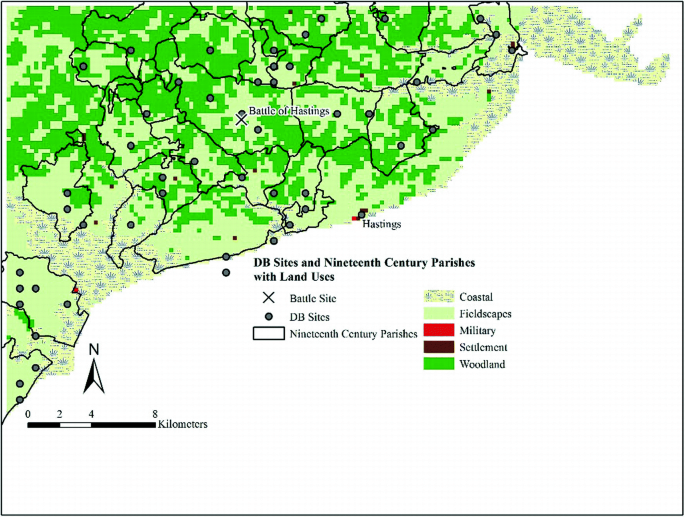The map depicts a detailed landscape focused on the Hastings area, highlighting historical and geographical elements. The coastline, extending from the top left of the image down to the center, is presented in pixelated shades of green, indicating different land uses. The water, mostly on the right and bottom edges, is depicted in white. The map prominently features an 'X' marking the Battle of Hastings towards the center, while Hastings itself is labeled near the bottom right.

Black dots signify DB sites, and white rectangles outline 19th-century parishes. The legend at the bottom explicates these symbols along with additional designations: light green for fieldscapes, red for military areas, black for settlements, and bright dark green for woodland. A north arrow is located at the bottom, near a scale in kilometers (0, 2, 4, and 8 kilometers), ensuring accurate distance measurement. Counties or provinces are delineated with various outlined shapes, providing further geographical context.

The map serves as an informative depiction of the historical landscape of Hastings, using specific symbols and colors to represent different areas and land uses effectively.